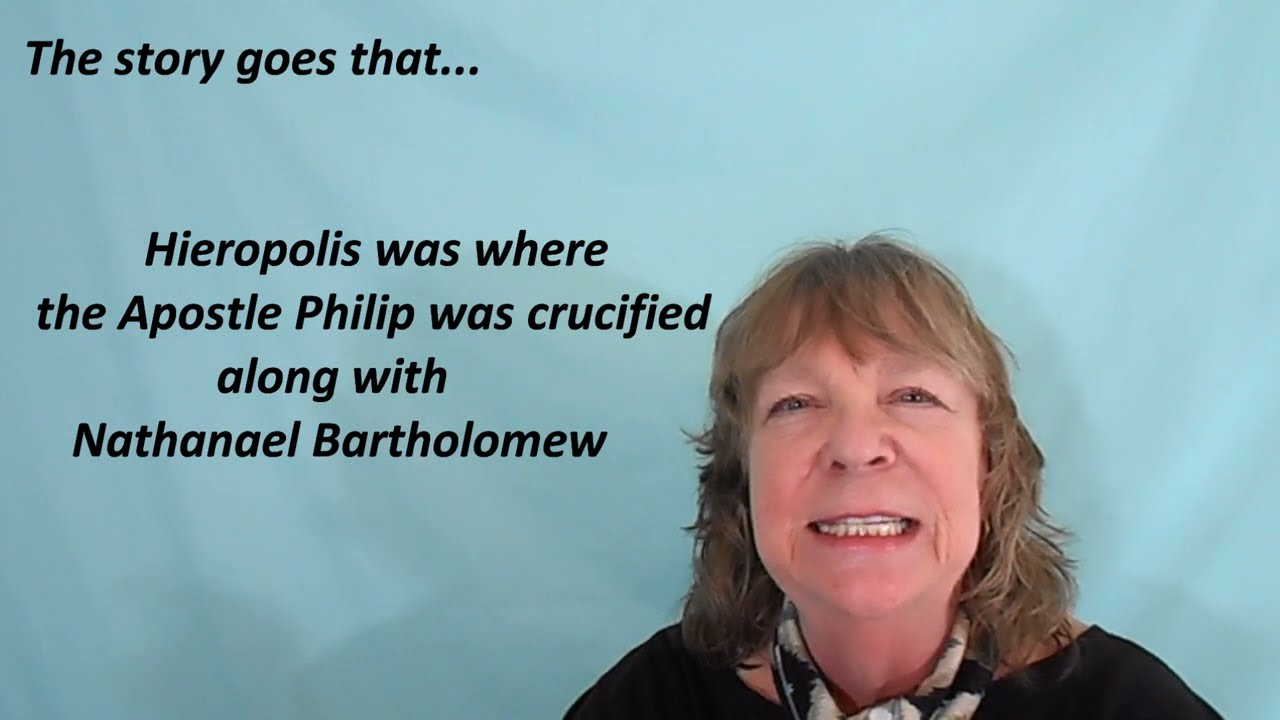The image is a screen grab from a video, depicting a middle-aged woman, likely in her mid-60s, positioned in the bottom right corner, with the image cut off just below her shoulders. She has shoulder-length, wavy brown hair and light-colored eyes. She wears a scarf around her neck and a black blouse. The woman's face shows an exasperated expression, akin to being captured mid-sentence, with her mouth slightly open, revealing both her top and bottom rows of teeth. The background behind her appears to be a light textured blue, possibly indicating the use of a green screen. In the top left corner of the image, there is a caption in black text that reads: "The story goes that Hieropolis was where the Apostle Philip was crucified along with Nathanael Bartholomew," suggesting the video discusses a religious topic related to biblical events.